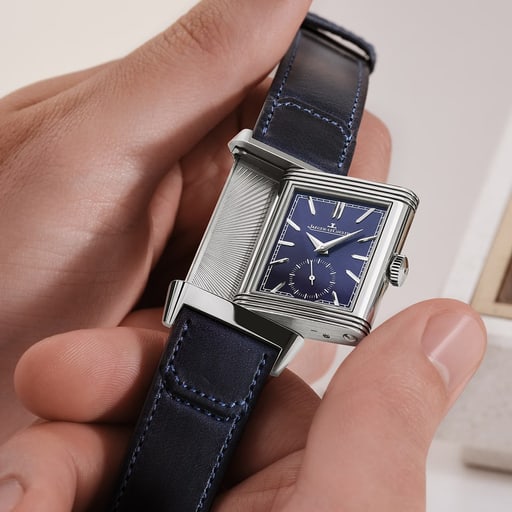In this detailed image, we see a close-up of a wristwatch being carefully examined by a pair of light-skinned hands. The watch itself has an almost square, slightly rectangular, silver face framed by a silver border. The face of the watch is a dark navy blue, featuring sleek silver lines in place of numbers, along with silver hour, minute, and second hands. This unique watch design allows the face to slide out partially from its position, suggesting possible reversible or interchangeable functionality. The band is composed of black leather with blue stitching, enhancing the watch's sophisticated appearance. The background is a light gray wall with a window that has a white and tan trim. The image, with its square shape, captures the careful manipulation of the watch, highlighting intricate details of the watch's design and craftsmanship.